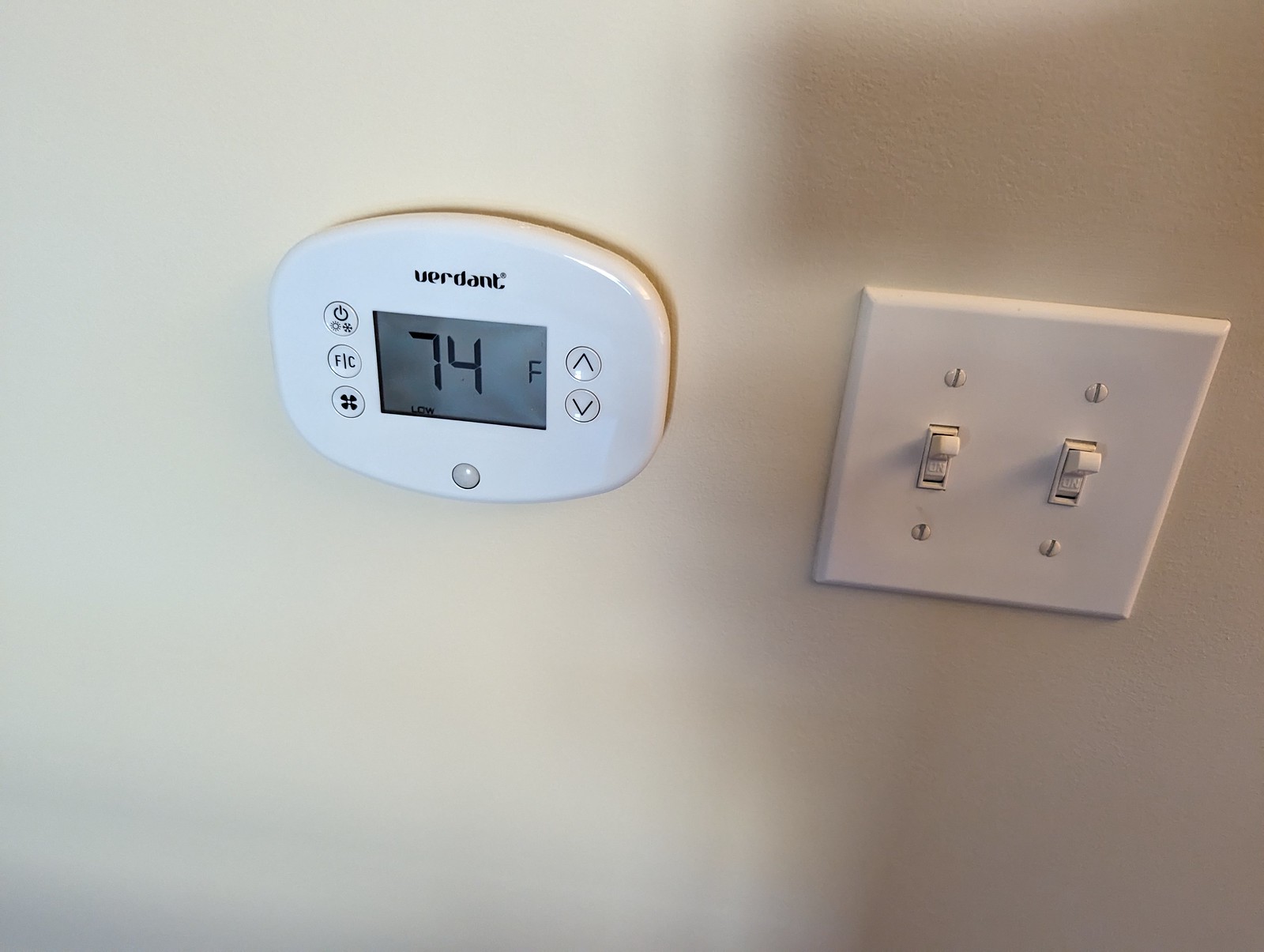In the photograph, a pristine white wall serves as the backdrop for two distinct objects positioned side by side. To the left is an advanced thermostat for an air conditioning and heating unit. This thermostat features a sleek, slightly rounded square design and is currently set to 74 degrees Fahrenheit with the fan speed on low. The control interface includes three buttons on the top left: a power button, a F/C button for switching between Fahrenheit and Celsius, and a fan button. To the top right, there are two arrow buttons for adjusting the temperature up or down. Above the digital display that shows the temperature, the brand name "Verdot" is prominently displayed. Below the display, there is a single round button.

To the right of the thermostat, there is a double light switch panel with four screws securing it in place. Both switches are in the off position. The white light switch panel casts subtle shadows on the wall, both above and below it, enhancing the sense of depth in the image. Both the thermostat and light switch blend seamlessly with the white wall, creating a minimalist and orderly appearance.